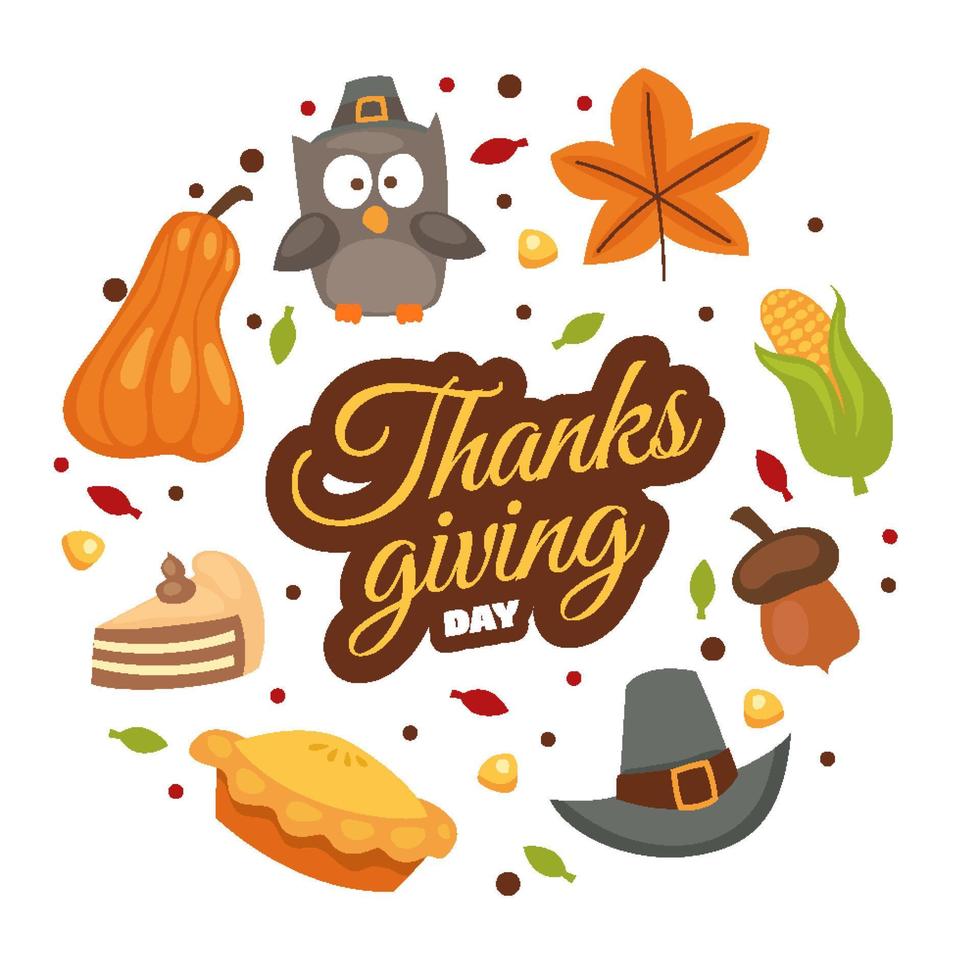This piece of Thanksgiving-themed clip art, ideal for classroom decoration, features a circular design set against a white background. At the center, the words "Thanksgiving Day" are prominently displayed in yellow letters on a brown backdrop. Encircling the central text, the illustration showcases various holiday icons arranged like the hours on a clock. Starting at the 12 o'clock position, there is a little gray owl wearing a pilgrim's hat, followed by an orange maple leaf, an ear of corn, a brown acorn, a traditional gray pilgrim's hat, a pie, a slice of chocolate cake, and a pumpkin or gourd. Scattered among these primary images are additional seasonal elements such as red and green leaves, golden acorns, and small brown and red dots. The overall color palette consists of warm fall shades, including yellow, orange, green, brown, and gray.